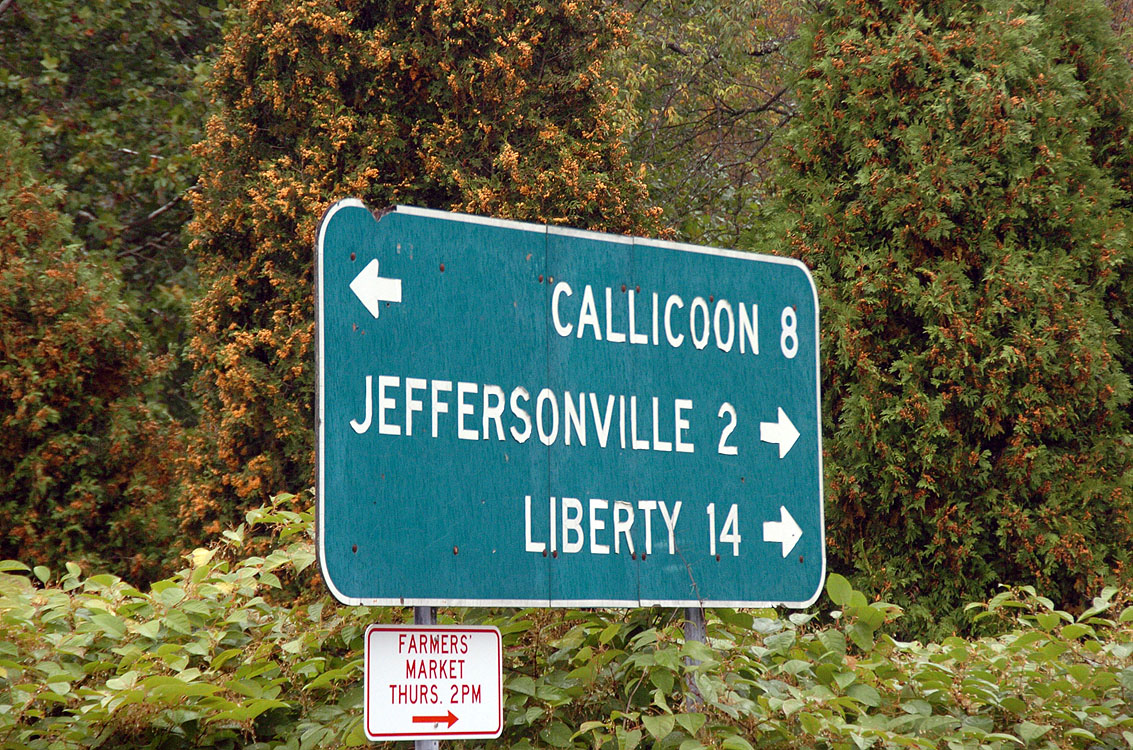This is a vibrant color photograph featuring a street sign set against a clear blue sky. The prominent, large rectangular sign has a thin white border and slightly curved edges. In the upper right-hand corner, "Calicoon 8" is written in white text. To the left of this text, there is a small white rectangle with a white arrow pointing to the left. 

On the next line down, "Jeffersonville 2" is displayed on the left-hand side, accompanied by a white arrow pointing to the right on the right-hand corner. Below this, "Liberty 14" is shown towards the right, with a white arrow pointing to the right. 

Beneath the main sign, a smaller white sign bordered in red features red text that reads "Farmers' Market, Thursday 2pm," accompanied by a red arrow pointing to the right. Surrounding the base of the signs are lush green shrubs, and in the background, taller trees with a mix of orange and green leaves can be seen, adding a touch of autumnal color to the scene.